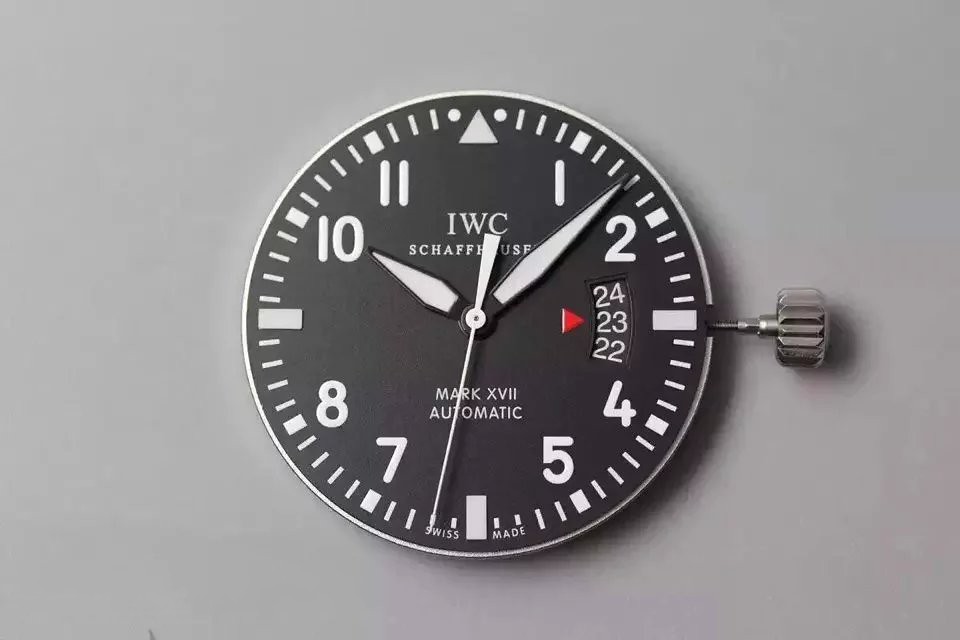The image depicts a large clock mounted on a light orchid-colored wall. The clock features a sleek design with a silver frame encircling a black face. White numerals are displayed at the 1, 2, 4, 5, 7, 8, 10, and 11 o'clock positions, while the 3, 6, and 9 o'clock positions are marked by simple silver squares. The 12 o'clock position is uniquely marked with a silver triangle. The clock's hands, including an additional second hand, are all silver. Additionally, a small red triangle indicates the date, pointing to the 23rd. The words "IWC" are inscribed in silver letters, alongside "Schaefer House" and "Mark XVIII Automatic." A noticeable crown, used for adjusting the time, is positioned on the side of the clock.